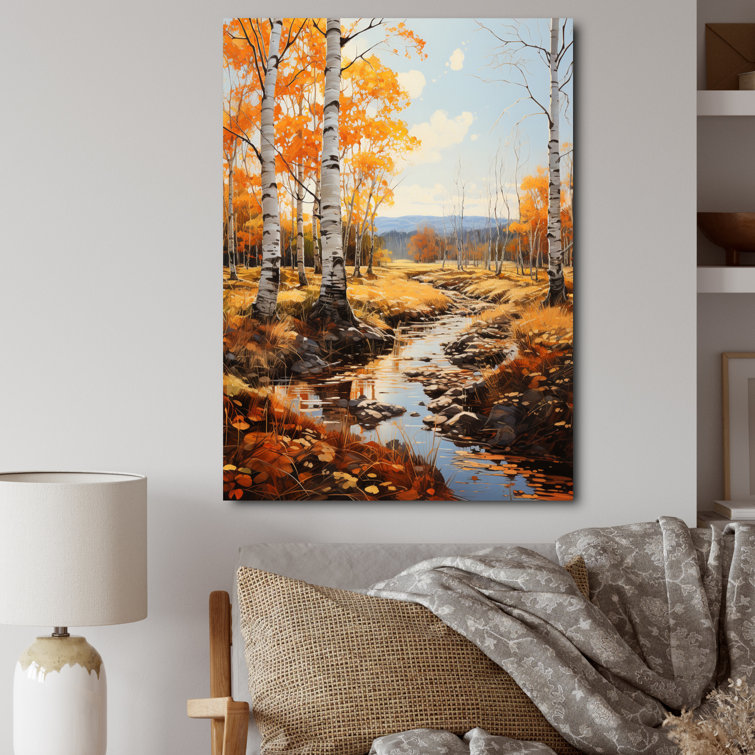This photograph captures a cozy living room or den, featuring a modern rustic couch with a thin wooden frame, brown burlap pillows, and a grayish-white throw draped over it. Adjacent to the couch is a table adorned with a lamp that boasts a pottery-style base and a plain white round shade. Although the table itself isn't visible, the lamp stands out with its off-white appearance, illuminated by natural daylight filtering into the room. Above the couch, a striking fall-themed painting dominates the wall: it showcases a vibrant landscape with a brook weaving through a forest of birch trees with white, gray, and black bark. The trees are adorned with orange and yellow leaves, set against a backdrop of a mountainous range under a bright blue sky dotted with clouds. To the right, built-in bookshelves provide additional character to the space, merging functionality with the inviting, rustic aesthetic of the room.